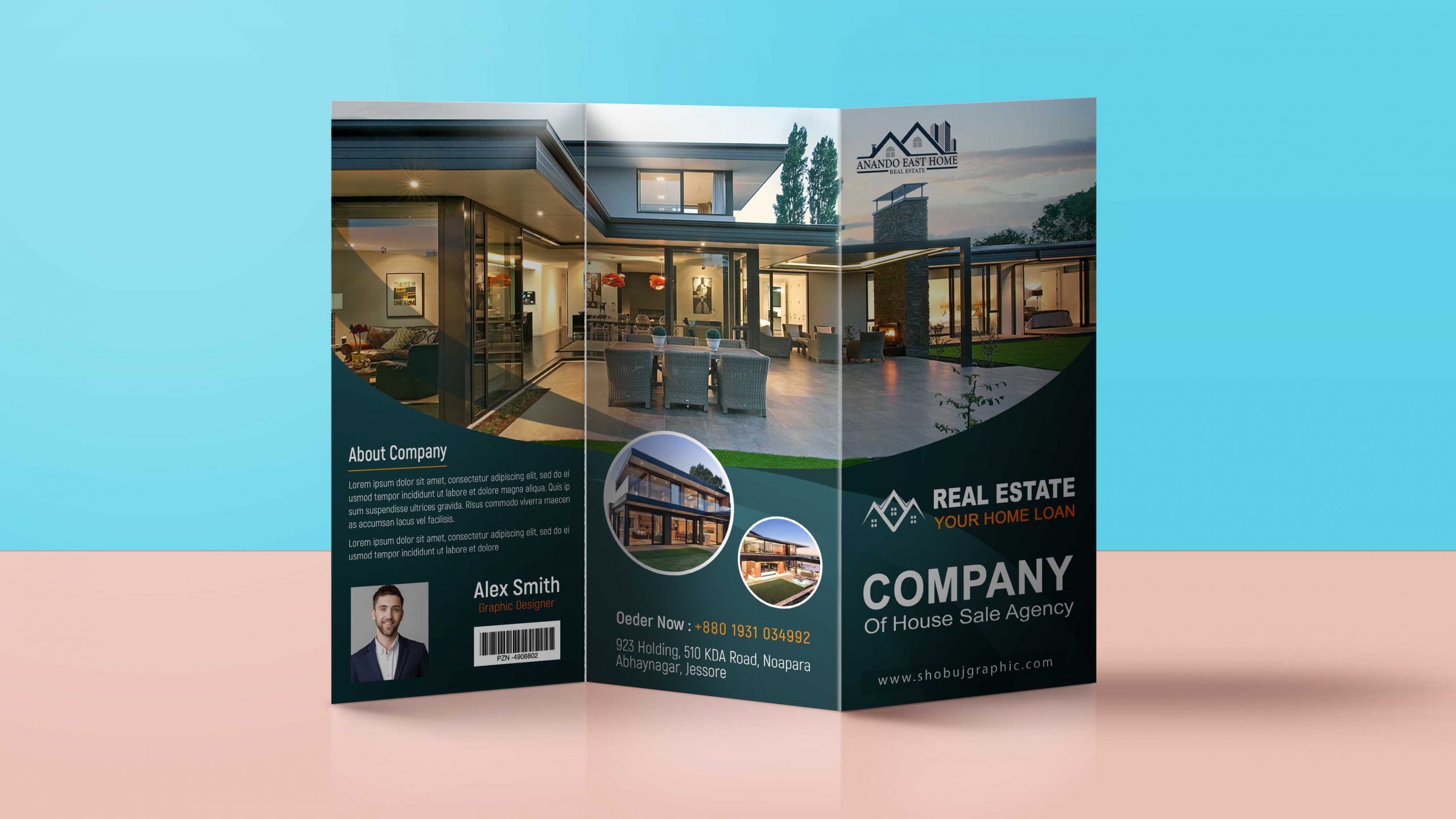The image shows a trifold brochure standing upright on a peach or light pink surface, against a background of sky blue. The brochure is an advertisement for a real estate company named "Anando East Home." The top part of the brochure features a name and logo, prominently stating "Real Estate, Your Home Loan Company of House Sale Agency."

The brochure displays several detailed images of a modern, contemporary two-story house with large floor-to-ceiling windows and an expansive stone patio. The middle panel includes two circular insets showcasing different views of the home. The brochure is divided into three panels, with text across all three at the top showing a continuous patio scene of the luxurious house.

On the lower left-hand corner of the brochure, there is a photo of a man named Alex Smith, presumably a realtor, alongside a barcode. One of the panels features a section titled "About the company" with additional details about the business, although some of the text is hard to read. The front panel also contains contact information, including a phone number and an invitation to "Order Now."

Overall, the brochure uses a mix of colors including dark green, light green, tan, white, and black, with dynamic graphical elements giving it a polished look, suitable as a template for a real estate marketing material.